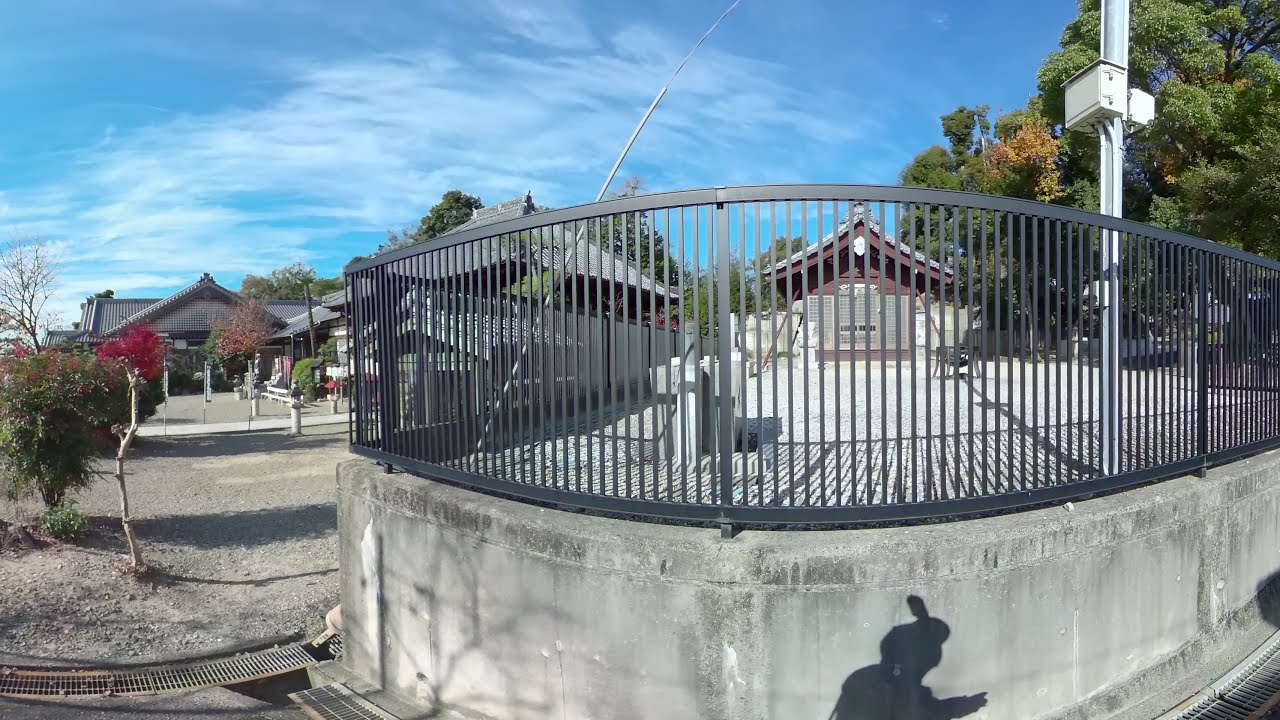In this outdoor scene, the image captures a picturesque view featuring a gated shrine reminiscent of East Asian architecture. On the left, a series of traditional buildings with dark brown, triangular rooftops stand at the back, supported by classic pillars. In front of these structures are various ornamental trees, some displaying a greenish-red hue, meticulously manicured and adding to the serene atmosphere. Near the bottom left of the image, a drainage system with small rectangular cutouts is visible on the ground.

On the right, an elevated platform or patio dominates, rising to the height of an average human head, and constructed on a gray foundation. This platform is encircled by a black wrought iron fence, which encloses a smaller shrine or temple with a gabled, slightly curved roof hinting at traditional East Asian design. A sign on a pole stands next to the fence, and a human silhouette is cast as a shadow on the concrete podium.

Surrounding the platform and stretching towards the left is an expanse of gravel or dirt, lined with posts and various shrubs, leading into a courtyard. This courtyard is enclosed on two sides by multiple wings of buildings, maintaining an archaic, classical architectural style, with a mixture of different colored shrubs and trees adorning the forefront. Overhead, the sky is a soft pale blue, interspersed with feathery white clouds, completing the tranquil and culturally rich tableau.